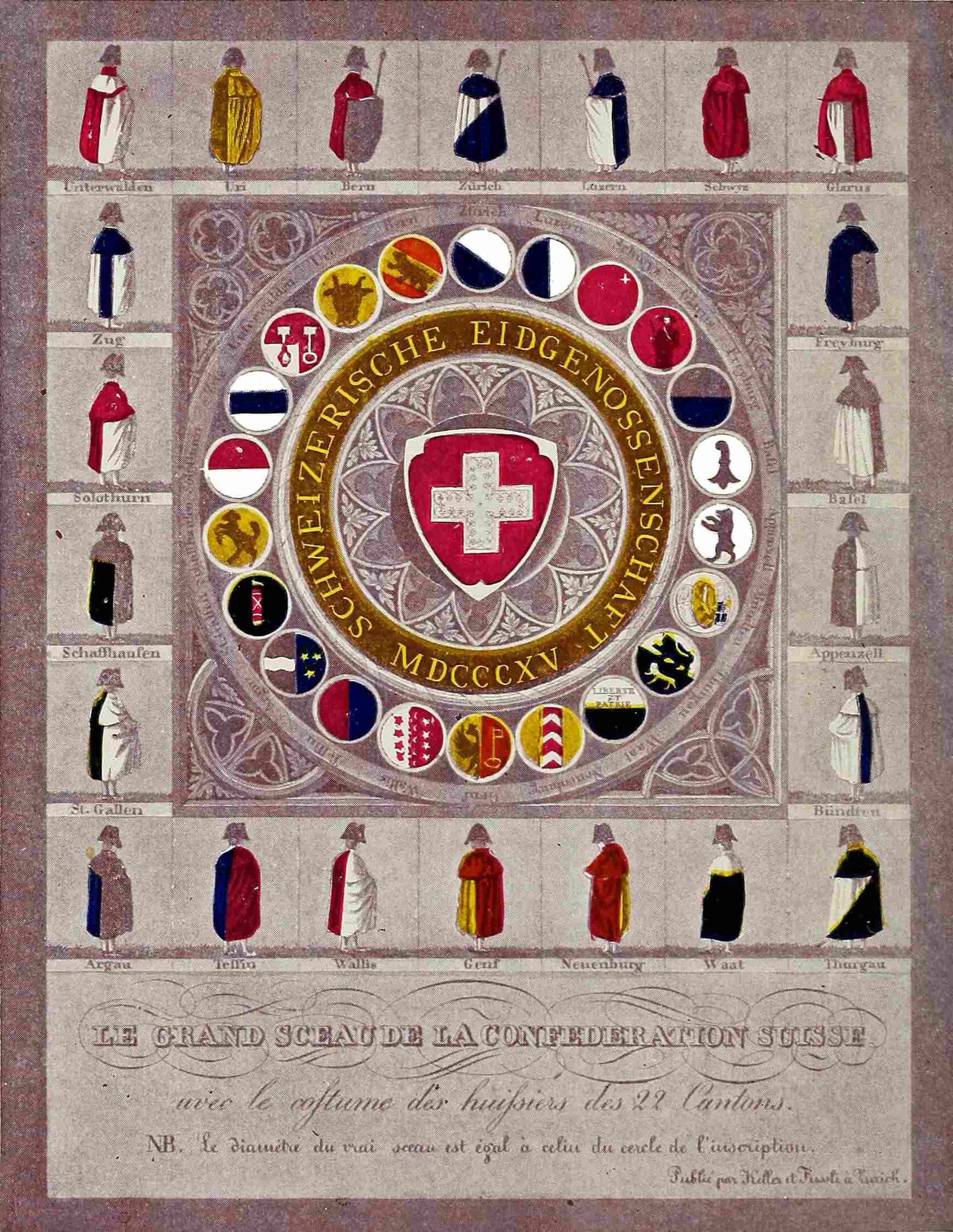The image appears to be of a detailed poster or wall hanging with a gray border around all sides. Inside, there is an arrangement of squares that form a frame, consisting of seven squares across the top and bottom, and six down each side. These squares each contain various images, likely of people in different types of clothing and gray hats, possibly adorned with shields or cloaks.

Centered within the square frame is a circular border in gray, embedded with various circular logos or symbols. This circular motif is again framed by an orangish border with yellow writing, possibly of German origin, reading "Schweizerische Eidgenosse." At the heart of the circle, there is a prominent shield with a red background and a white cross.

The people depicted within the square frame are dressed in a variety of colored gowns, including combinations of black, white, red, yellow, gold, and gray. These figures seem to be arranged in a grid and could be representing different heraldic or historical figures, possibly from Swiss history, given some context from the partially readable text.

At the bottom of the image, there is a long gray rectangle containing some hard-to-read text, which might indicate a title or further description. The overall image is clear and brightly lit, ensuring all elements are visible, even if the specific language and some finer details are hard to decipher.